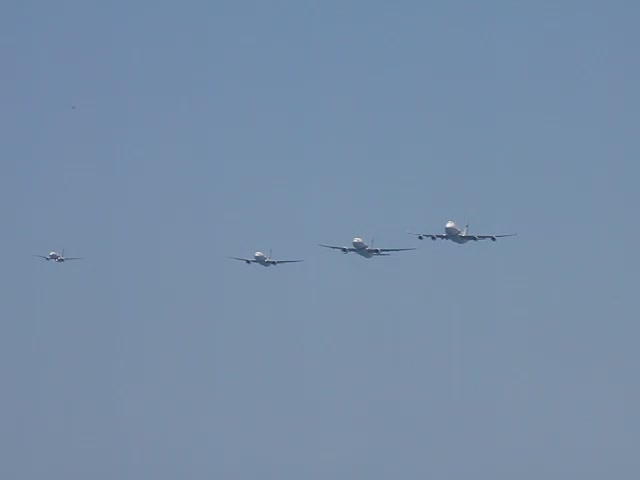In a beautifully clear, completely blue sky without a single cloud, this photograph captures four large airplanes in flight. The focal point is three planes flying in a parallel line towards the right side of the image; the one on the far right appears to be leading and is distinguishable by its four engines, while the two trailing it each have two engines. These planes, likely commercial airliners given their size and shape, demonstrate a subtle formation more evident due to their spacing and alignment. Positioned further to the left is another airplane, which is slightly smaller and somewhat isolated from the trio, yet maintaining a similar altitude. The bright, daytime setting makes for a perfect backdrop, highlighting the sleek, possibly white or gray fuselages of these high-altitude aircraft. The scene conveys a sense of majestic precision and calm in the open sky.